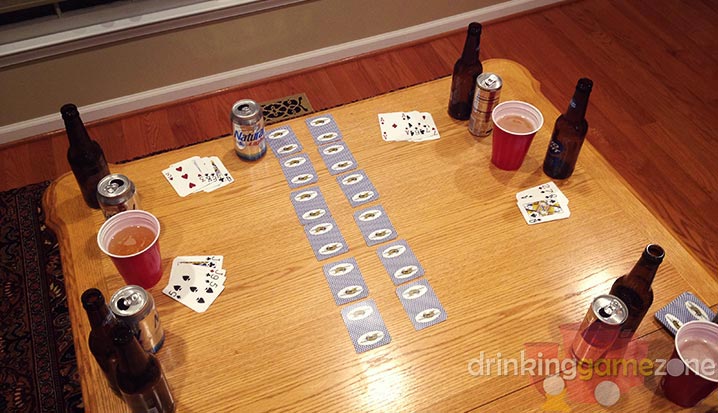The indoor setting features a dimly lit room with dark brown walls and cherry wood brown flooring, accented by a small floor vent and a rug. At the center stands a square table made of light brown wood, adorned with a variety of items that suggest a lively game night. Arranged around the edge of the table are several brown glass bottles, beer cans, and red solo cups, hinting at a gathering of friends. The tabletop is also scattered with playing cards; some are neatly arranged in rows, face down, while others are flipped open, ready for play. In the lower right corner of the image, a text overlay reads "Drinking Game Zone," indicating the playful atmosphere. This setting, with its carefully placed cards and drinks, evokes a sense of camaraderie and fun, perhaps even designed for an advertisement promoting a social gaming experience.